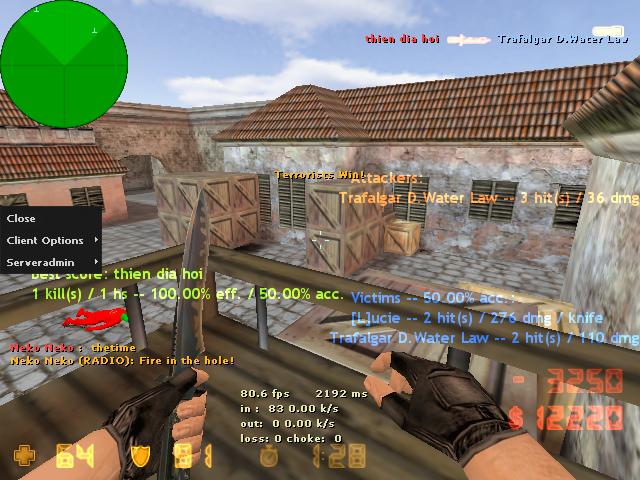This is a detailed caption for the image:

"A high-resolution screenshot captures an intense moment from a first-person video game, providing a view of an outdoor village scene. The player, represented by the hands of a Caucasian man adorned with black fingerless gloves, is equipped with a knife in his left hand, its blade pointed upward. The player's right hand is empty. He stands on a sturdy brown wooden platform, gazing over a cluster of rustic buildings partially obscured by several wooden crates. In the upper left-hand corner of the screenshot, a green circle likely signifies a navigational map or HUD element, aiding the player in orientation. Overlaid text on the image suggests active game development or real-time information updates, adding a layer of technical intrigue to the scene."